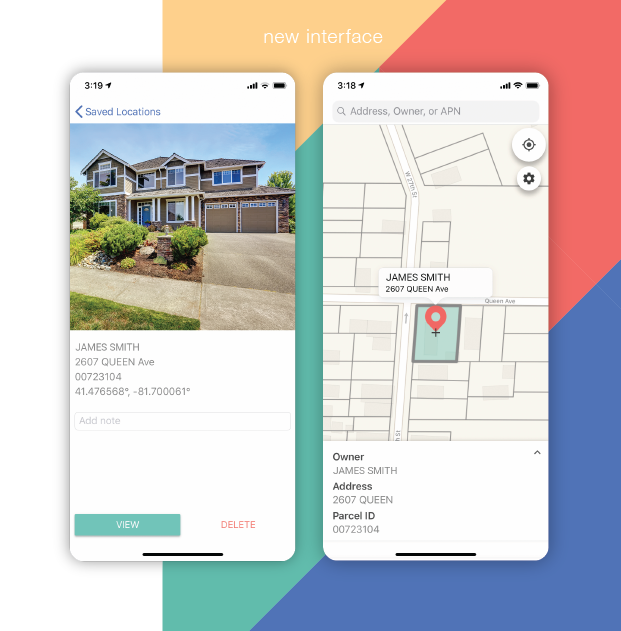The image features a side-by-side comparison of two elements: a detailed photograph of a house and a corresponding map. On the left side of the image, there's a picture of a two-story home with a two-car garage and numerous windows. Text below the photograph includes pertinent details: the name "James Smith," the address "2607 Queen Avenue," the parcel ID "00723104," and geographical coordinates "41.476568, -81.70061."

The right side of the image displays a map highlighting the location of the house with a marker. Similar information is provided here: the owner's name "James Smith," the address "2607 Queen," and the parcel ID "00723104." The map gives viewers a geographical context of the home's location.